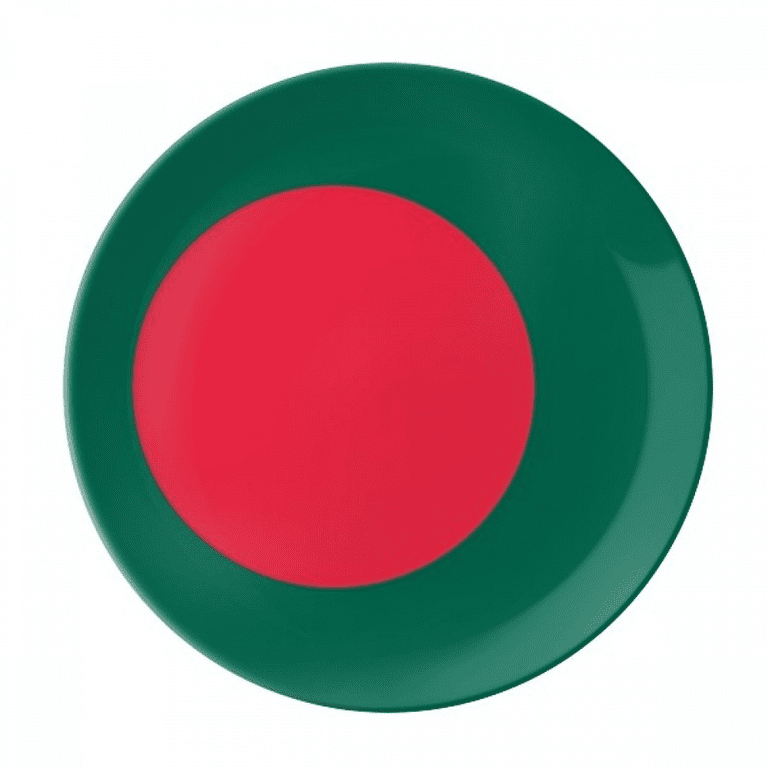The image appears to be computer-generated, depicting two concentric circles. The outer circle is a large, two-toned green circle, predominantly a dark forest green with a lighter spring green accentuating the edge, giving it a subtle shaded appearance. Inside this outer circle, slightly off-center to the left, is a smaller, solid bright red circle. The vibrant red contrasts sharply with the green, making the central circle stand out prominently. The absence of a background accentuates the vivid colors and simple geometric composition, emphasizing the relationship between the two differently shaded green tones and the striking red of the inner circle.